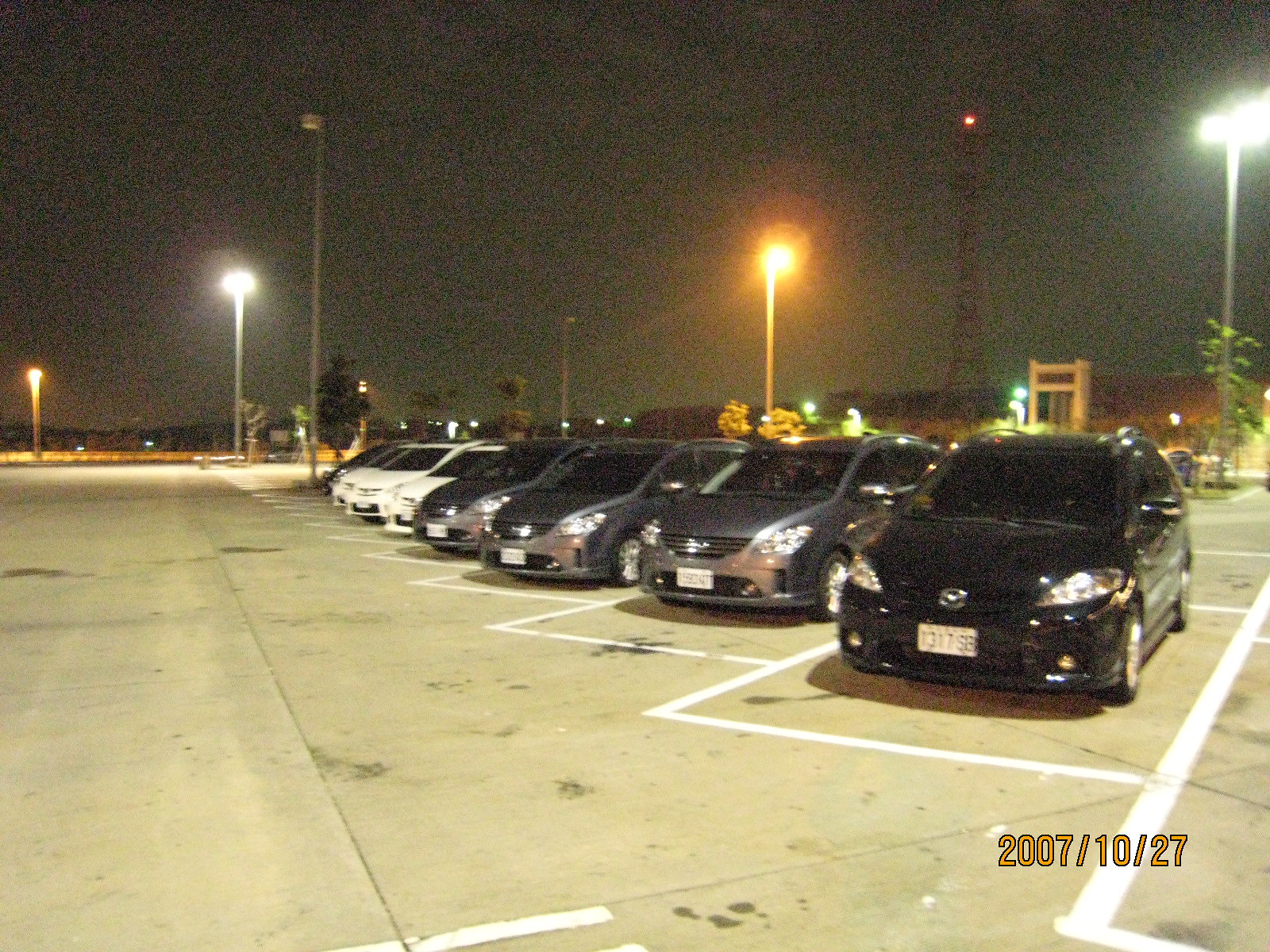This is a grainy, horizontal rectangular photograph taken at night, depicting a concrete parking lot lined with white parking spaces. The scene captures eight cars, all sedans, parked frontward and staggered, creating a single, uninterrupted row. The first car on the far right is black, followed by several gray cars, and then white ones further back. The picture gives the impression of a car rental company due to the similarity of the vehicles. Street lamps on tall steel poles illuminate the area with a mix of cold white and warm yellow lights. In the distant background, approximately one-third from the right-hand side, stands a tower reminiscent of the Eiffel Tower, marked with a red light at its pinnacle. Above, the sky is dark, emphasizing the nighttime setting. A date stamp in yellow lettering at the bottom right corner of the photograph reads "2007/10/27."